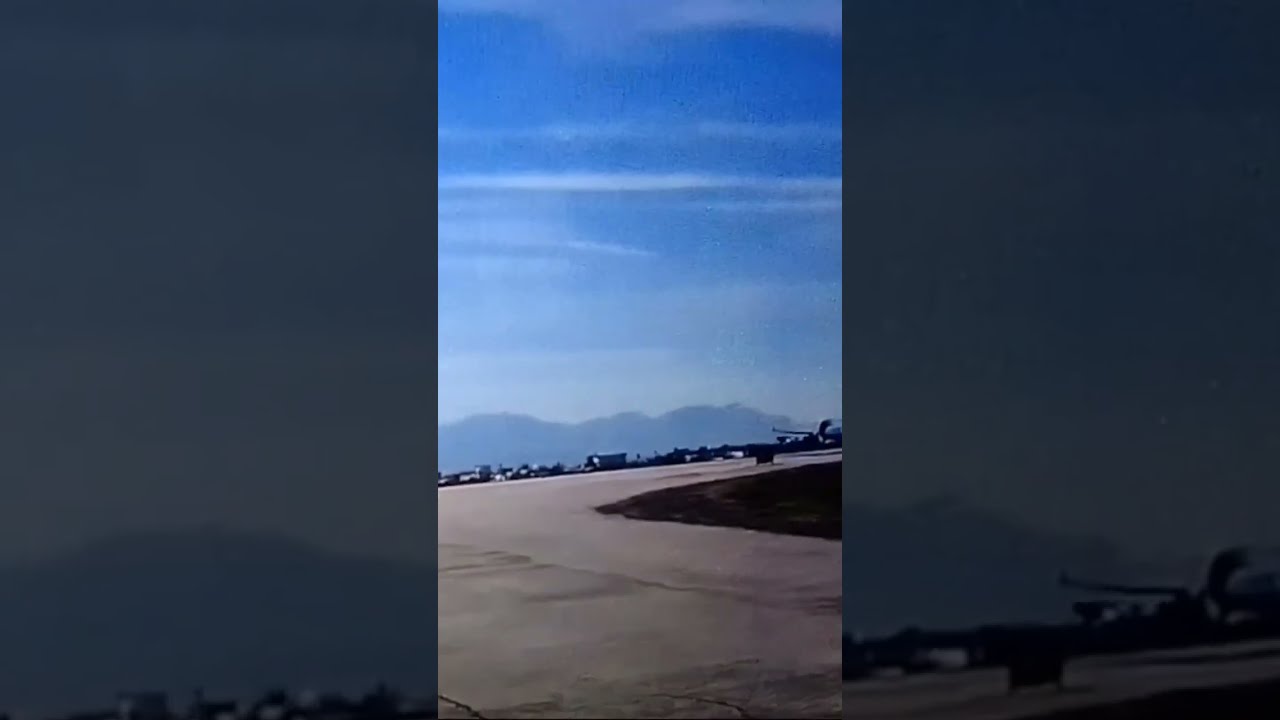The image showcases a blurred portrait screenshot from a video, centered on a curved, flat runway or airport tarmac. The right side of the image partially shows an airplane, possibly parked or preparing for takeoff. The foreground features a gray concrete pathway that lacks guard rails, leading potentially to a drop-off. There's a hint of grass patches near the bottom right, adding a slight touch of green. The background is dominated by distant, shadowy mountains, with a blue sky above dotted with thin, wispy clouds. On either side of the central image, darkened and enlarged versions of the same photo highlight details of the mountains and parts of the pathway, emphasizing the uniform composition. The image uses a palette of blue, white, gray, dark green, and brown tones.